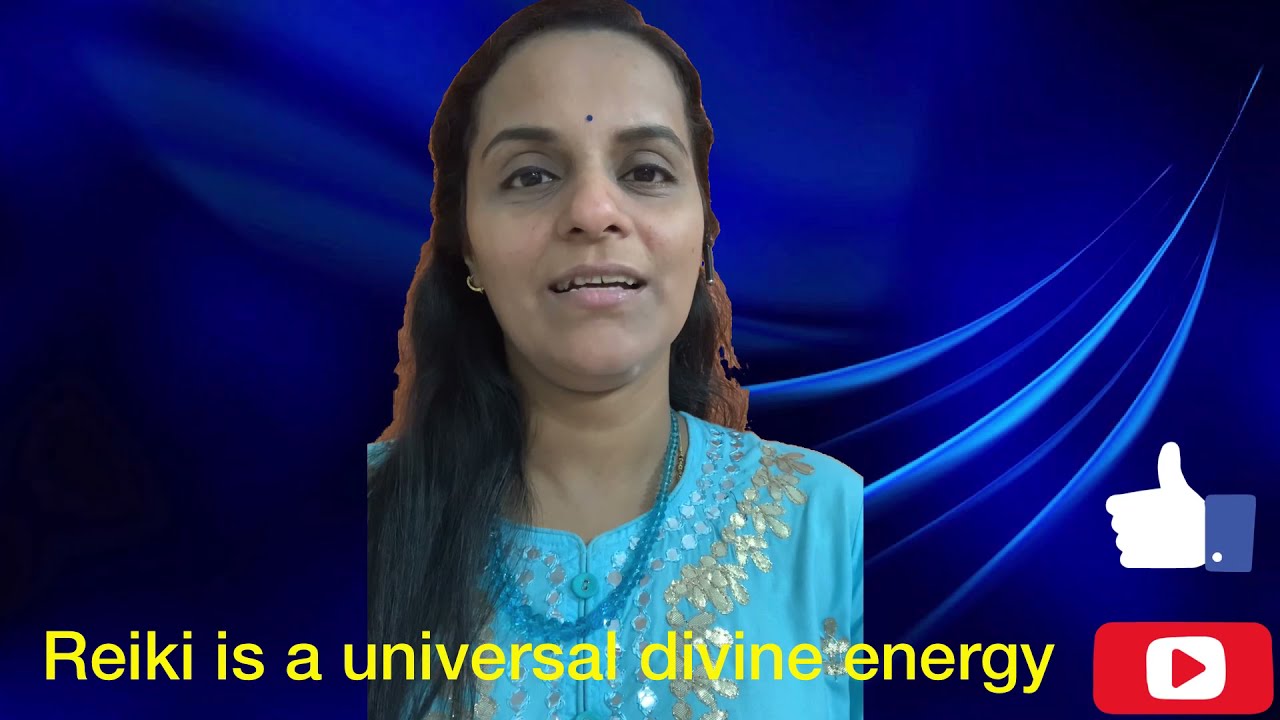This image is a screenshot from a YouTube video featuring an Indian woman with long brown hair, partially tied with a hair accessory, wearing a light blue blouse adorned with gold embroidery and sporting a matching blue necklace. She is seen from the shoulders up, seemingly in the middle of speaking, with her mouth slightly open. Her attire includes earrings and a bindi-like black dot on her forehead. The background is a digitally overlaid design with deep blue tones and lighter blue streaks originating from the top right corner, expanding towards the center. The bottom right corner features the YouTube logo and a thumbs up icon, indicating it's a YouTube video. Yellow text across the bottom states "Reiki is a universal divine energy," possibly reflecting the video's subject matter. The woman’s image takes up most of the frame, emphasizing her as the main focus of the screenshot.